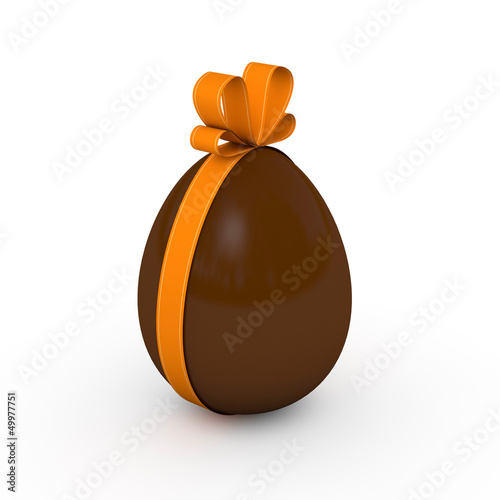The image is a stock photo, identified by the Adobe stock pattern repeated diagonally across it and the text "Adobe Stock" with the stock number 49977751 written vertically in small black font at the bottom left-hand corner. The central feature is a vertically positioned chocolate egg wrapped elegantly with an orange ribbon tied into a neat bow at the top. The ribbon extends around the egg's longest side, with the bow displaying intricate detailing where the middle two loops are larger compared to the smaller outer loops. The egg features subtle shading near the bottom and within the bow’s ruffles, contrasted by a highlighted shine near the top. The background is completely white, enhancing the prominence of the chocolate egg and its decorative ribbon.